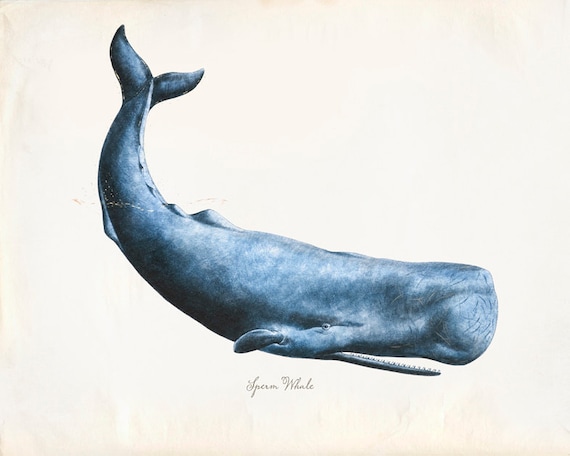The image is a highly detailed and well-rendered color drawing of a sperm whale against a beige background. The whale, identified by the cursive white script "sperm whale" at the bottom of the image, appears massive with its front positioned on the right side, extending back to a tail that curves upward, pointing towards the top of the image. The sperm whale is illustrated with a bluish hue, showcasing intricate details such as scratch marks across its thick head, highlighting its scars and texture. The open mouth reveals its teeth, and its small fins and powerful tail are accurately depicted. The eye, situated above the mouth and distant from the whale's tip, exudes a mournful expression. This remarkable drawing effectively captures the contours and highlights of the sperm whale's skin, emphasizing its majestic and somewhat rugged appearance.